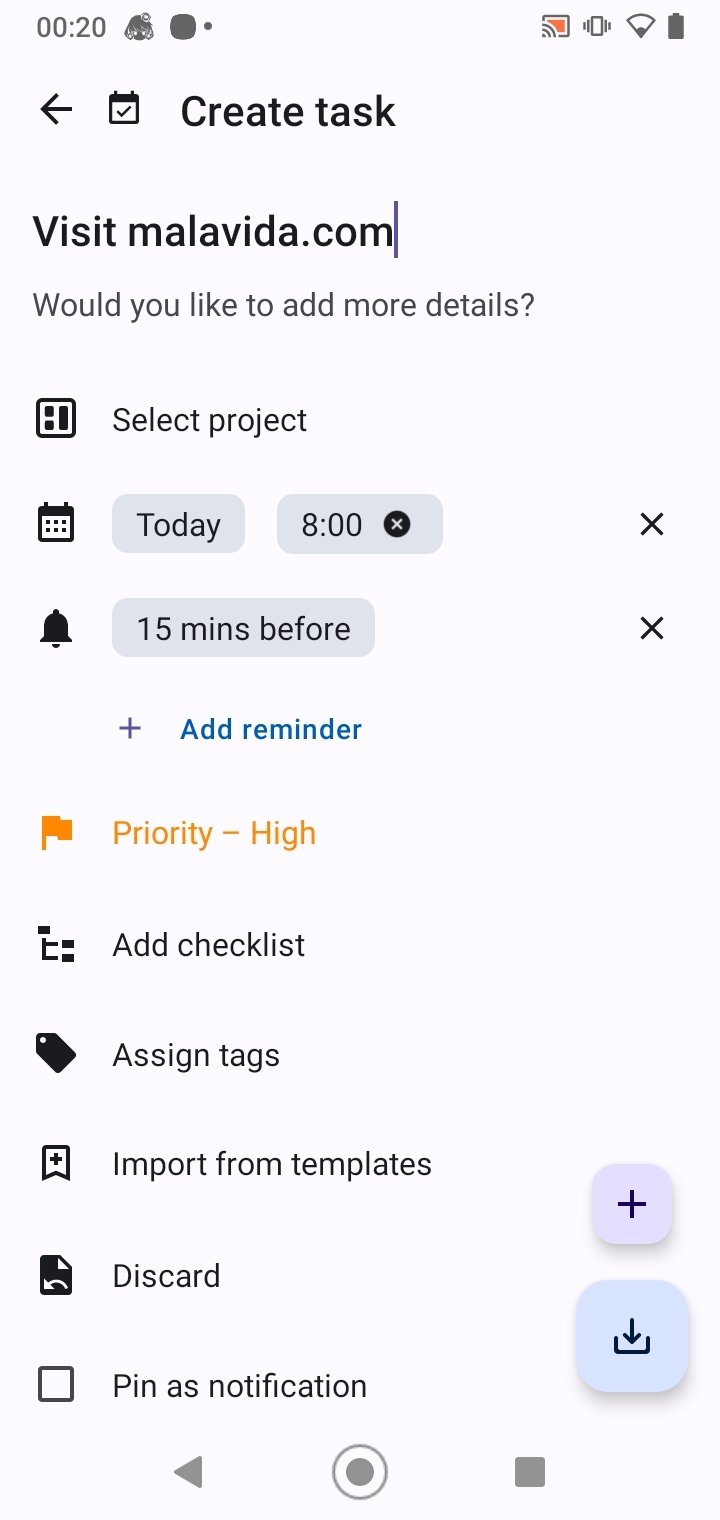Screenshot of a Phone Displaying a Task Management App:

The background of the image is white, resembling a screenshot taken on someone's phone. At the very top, there is a time reading "00:20". Below the time display, there is a gray interface featuring elements such as what looks like a gray face or door, a gray square, and a gray circle. On the right side of the gray interface is an orange and white rectangle, alongside different shades of gray patterns and a gray battery icon.

On the left side of the next row, a black arrow points to the left-hand side, followed by a black check mark and the text "Create Tasks" in black. Below this is some space and the text "Visit malavita.com" in black, along with a prompt asking, "Would you like to add more details?"

Further down, the app displays "Select Project" with two gray rectangles beneath it. The first rectangle is labeled "Today" in black, while the second one says "8.00" with a black circle featuring a white 'x' inside it. On the right, there is a black 'x' icon.

Underneath these fields, there is a line with a black bell icon and another gray rectangle labeled "15 minutes before" in black. This section is followed by another 'x' icon. Below these elements, a plus sign appears next to blue text that says "Add Reminder."

Further down, there is an orange flag with text "Priority - High" next to it. In black text, it says "Add Checklist," and below that, "Assign Tags" is indicated with a black tag icon. Following this, there is a plus sign inside a band with the text "Import Templates." At the bottom of the image, there is an icon for Discord, with the option "Pin as Notification" displayed.